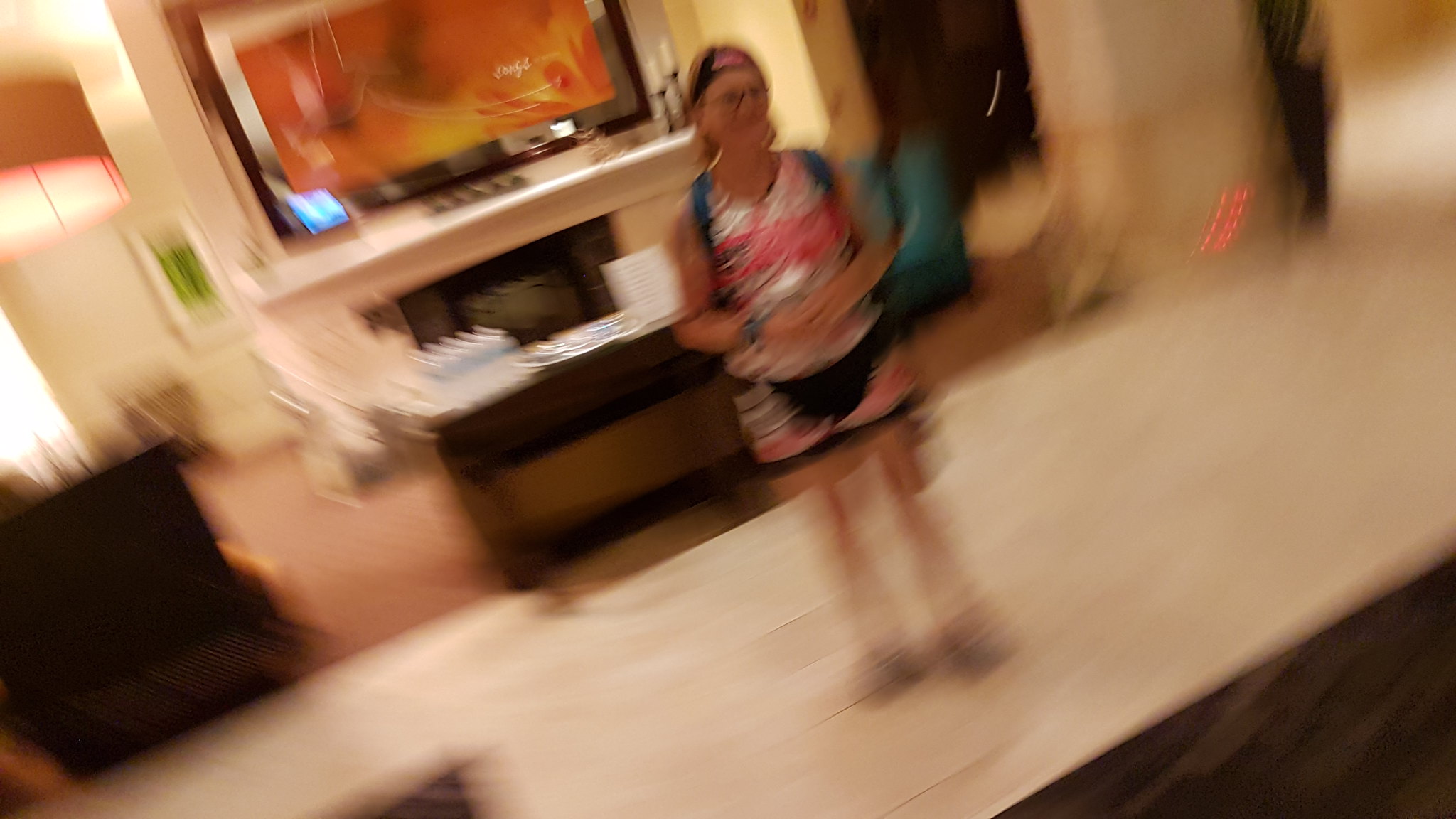This photograph captures a dynamic scene in what appears to be either a living space or a hotel room, characterized by an intriguing motion blur that adds a swirling effect to the colors, converging to the left. The individual in the foreground is wearing glasses, a headband, a tank top, and shorts featuring a striking pattern of white, black, and pink. They also seem to be carrying a backpack, as suggested by the visible blue straps, and may be wearing a wristwatch, although its details remain indistinct due to the blur.

The room's background is a blend of stylish and functional elements. Dominating the wall is a large television encased in a silver frame, displaying an orange-hued image. Below the TV is a white mantled fireplace that adds a touch of elegance to the setting. A blue chair is slightly visible towards the rear, surrounded by brown tables. The floor features what appears to be a white rug, though it could be another type of flooring due to the lack of clear detail. The scene is completed with reddish-brown carpeting, contributing a warm and cozy atmosphere to the room.